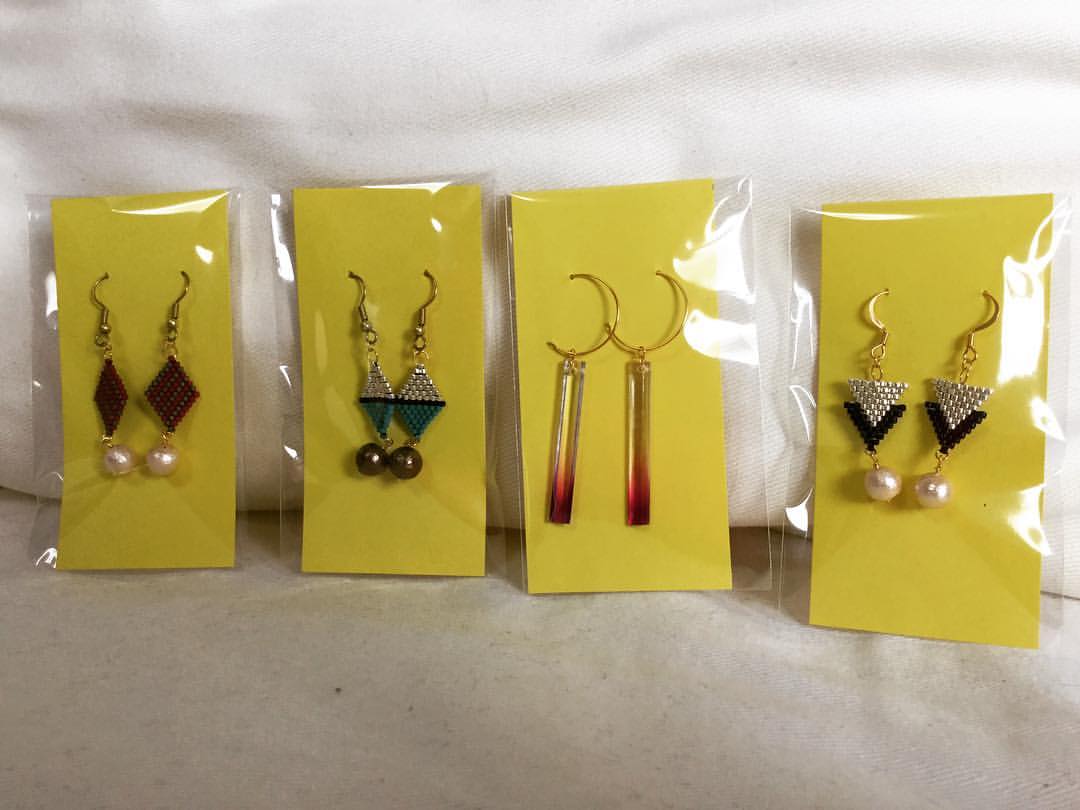The image showcases a detailed and well-organized photograph of four different pairs of earrings, each still in their original packaging. These earrings are attached to bright yellow cards and enclosed in small plastic bags, presumably for an online listing. The background consists of a soft, white, pillowy fabric, suggesting a cozy or aesthetically pleasing setting, possibly a blanket.

Starting from the left, the first pair features diamond-shaped earrings made of bronze materials. They are striped diagonally and adorned with little red beads, ending with a dangling pinkish pearl. 

The second pair consists of dangly earrings with gold-toned clasps and a diamond shape. The top part of the diamond is silver while the bottom is teal. These earrings also feature a darker-toned brown pearl hanging underneath.

Moving to the third pair, these earrings are notably different, distinguished by their very long rectangular shape. Made of a clear material that fades into crimson red at the bottom, they are strikingly elegant. Each earring starts with cylindrical yellow tops transitioning to red at the bottom.

The fourth and final pair features an arrangement of two overlapping triangles. The top triangle, pointing down, is silver and positioned on top of a black triangle. These earrings are finished off with a dangling white pearl bead, adding a classic touch to their modern design. 

Overall, the image conveys a clear and organized visual of the earrings, emphasizing their unique designs and consistent packaging presentation.